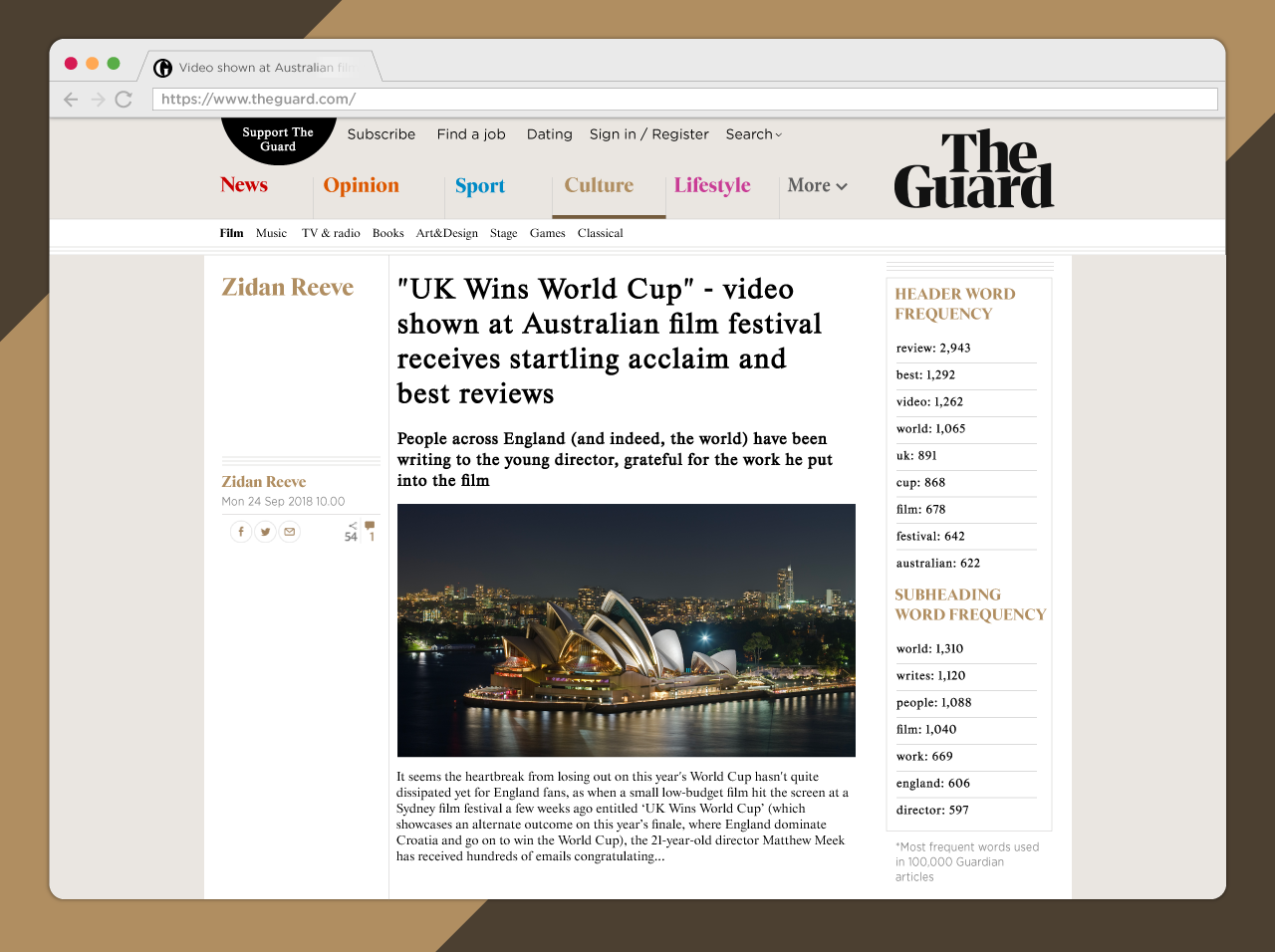The image depicts a webpage with a search bar at the top displaying "www.theguard.com." Below the search bar are navigation options in various colors: "News" in red, "Opinion" in yellow, "Sport" in blue, "Culture" in brown (and underlined), and "Lifestyle" in pink. To the far right, in black text, is "The Guard." 

Underneath this header, on the left, appears a headline in gold or brown text: "Zidden Reeve, 'UK wins World Cup.'" A subheadline reads, "Video shown at Australian Film Festival received startling acclaim and best reviews. People across England and indeed the world have been writing to the young director grateful for the work he put into the film."

The image also prominently features the iconic Sydney Opera House in Australia, recognizable by its tall, arching shapes and surrounding lights.

In the top right corner of the image are the texts "Header Word Frequency" and "Subheading Word Frequency," suggesting a focus on analyzing the frequency of words used in webpage headers and subheadings. 

The background transitions from a darker brown in the left corner to a lighter tan in the center, giving the image a dynamic, visually appealing gradient.